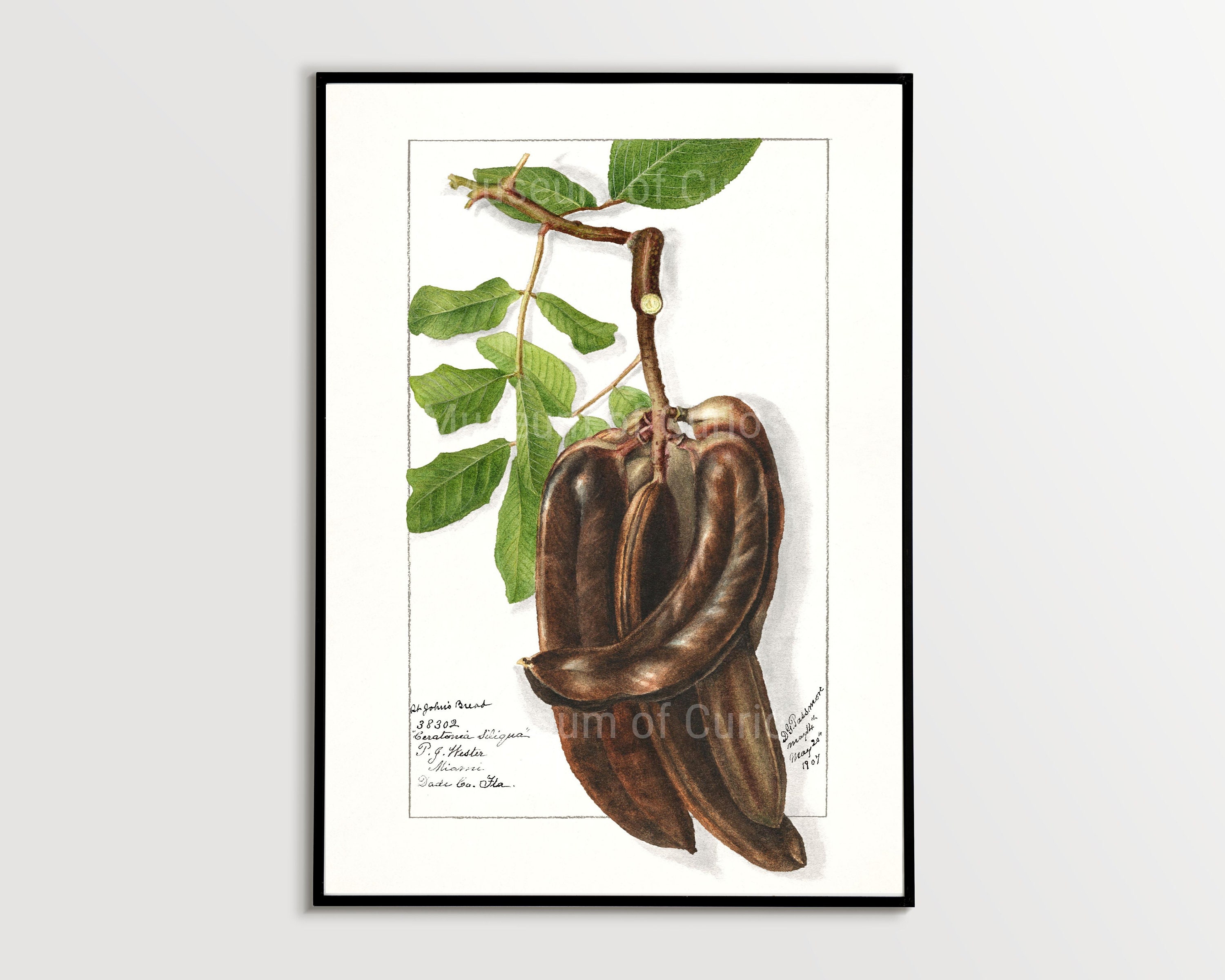The image is a finely detailed art piece, displayed vertically on a basic white wall. The artwork is rectangular and encased in a thin black frame, featuring a large matte white border integrated into the design. Within the white matte, there is a thin black line forming an inner square, out of which a plant emerges. The plant resembles a banana or plantain tree, with a prominent brown stem from which several brown, sharp-edged, and pointy fruits hang. Despite their shape reminiscent of bananas, they appear very dried up. Above, the main branch arches to the left with thin offshoots that bear vivid green leaves, providing a contrasting lively touch against the dry fruits. The entire composition has a very animated quality and includes a watermark, indicating a level of sophistication often associated with professional artwork.